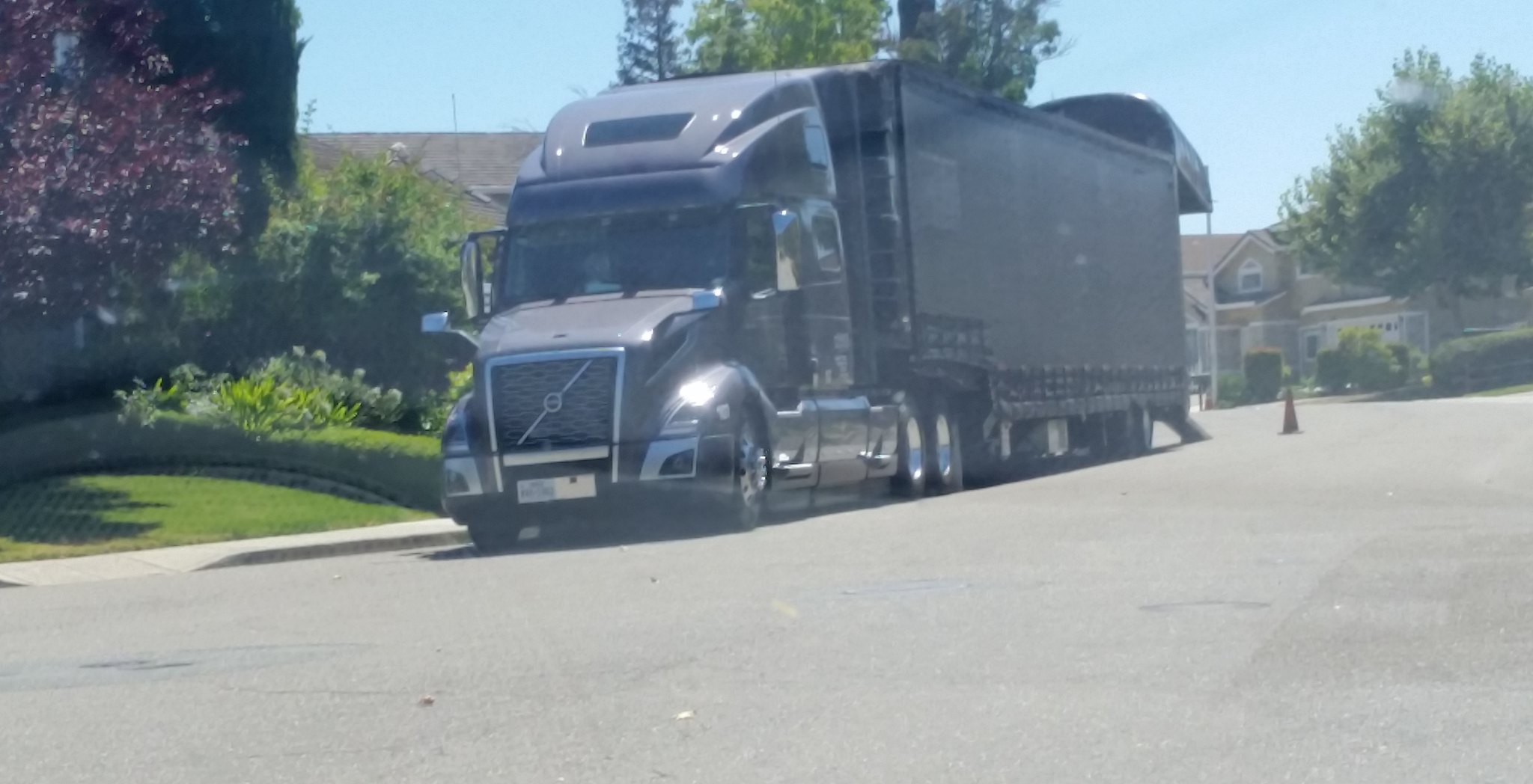This photograph captures a gray 18-wheeler big rig truck parked on the side of a well-maintained residential street, possibly in front of an apartment complex or cluster of well-appointed homes. The truck's ramp is extended at the back, suggesting it may be facilitating a delivery or move, indicated also by an orange safety cone placed near the street. The street itself features a lighter gray pavement, complementing the truck's color. Surrounding the scene, lush greenery flourishes, including professionally landscaped lawns, sculpted bushes, a variety of flowering plants, and several trees—one of which boasts vibrant violet leaves amidst the predominantly green foliage. The sky is clear blue, reinforcing the image's summertime setting. The atmosphere is serene, with no other vehicles or people in sight, highlighting the tranquility and orderliness of this picturesque neighborhood.